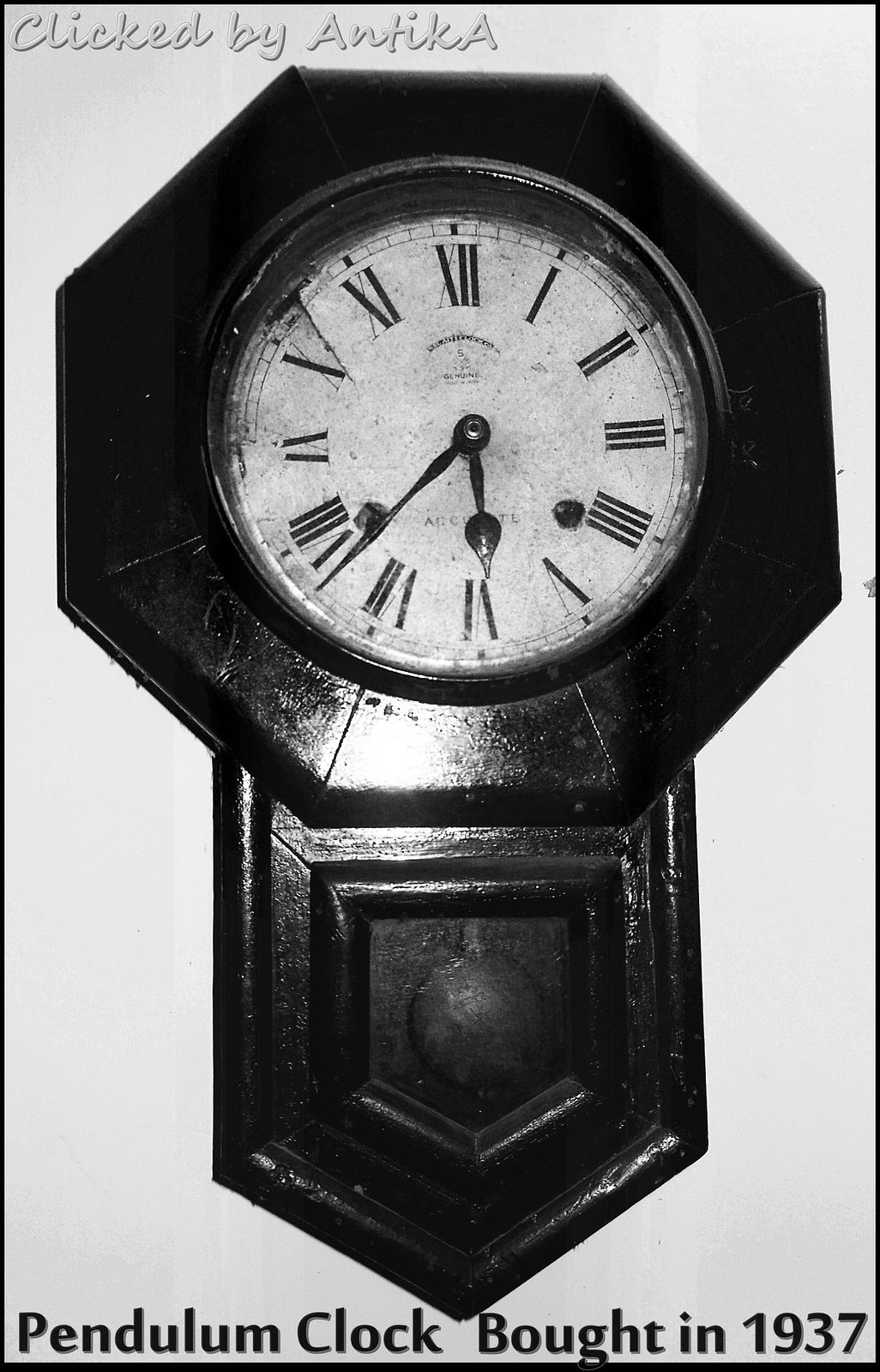A vintage black and white photograph prominently features a classic pendulum clock. In the upper left corner of the image, modern text credits the photo to "Clicked by Antica," suggesting the image may have been sourced from Pinterest. At the bottom, vintage black text reads, "Pendulum Clock, bought in 1937," providing context and a touch of history. The clock itself boasts elegant Roman numerals on a white clock face, indicating the time as approximately 6:40. Encased in a robust wooden frame, the clock's pendulum is visible swinging behind it. The photo evokes a sense of nostalgia and timeless craftsmanship.